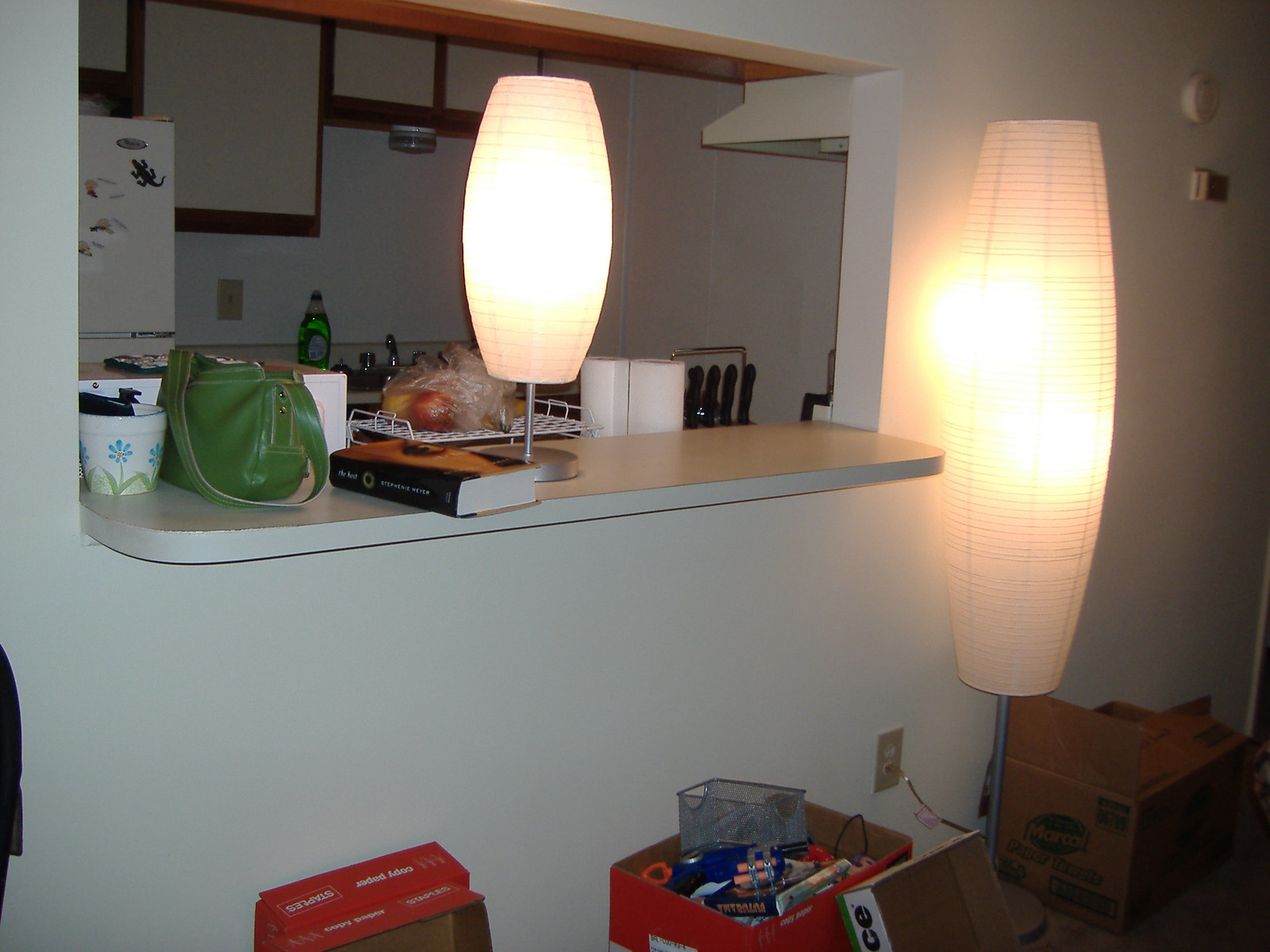The rectangular photograph showcases a residential home's bar area seamlessly transitioning into the kitchen. The dominant color theme is white, offering a clean, contemporary look. Starting from the top left corner of the image, there's a cutout in the wall that visually connects the bar area to the kitchen. Positioned on the bar counter below, which is also white, is a table lamp with a cylindrical lampshade. The lamp features a single silver metal pole attached to a round base, centered on the counter. Adjacent to the lamp is a book with a striking black cover, displaying a zoomed-in image of someone's face. To the left of the book lies a green leather handbag, adding a pop of color to the otherwise neutral setting.

Peering through the cutout in the wall, the kitchen presents a continuation of the white aesthetic. In the top left corner stands a white refrigerator, and below it, white cabinets with brown trim are visible, contributing to a slightly rustic touch. The walls in the kitchen, like the bar area, are painted white. A portion of the sink is in view, marked by a curved stainless steel faucet with two knobs flanking its sides. Right next to the sink, a clear plastic bottle of green soap detergent is noticeable, indicating a practical, lived-in space. The photograph effectively captures the blend of style and functionality in this residential environment.